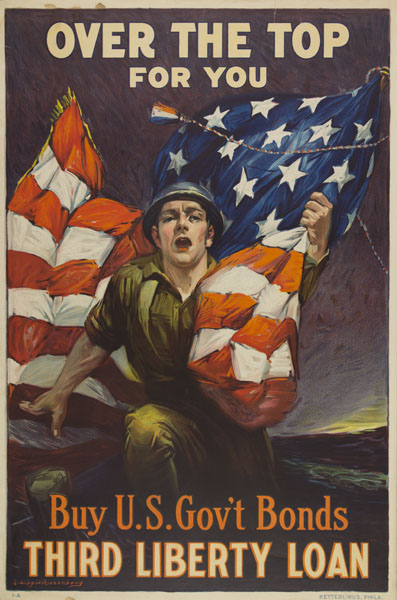The image depicts a vintage World War II recruitment poster for U.S. government bonds, done in a classic propaganda style. At the very top of the vertically oriented poster, in cream-colored letters, it reads "Over the Top for You." Below this header is a dynamic illustration of a young white male U.S. soldier, probably in his early 20s, charging forward. He is depicted wearing the customary military attire, consisting of khaki pants, a khaki shirt with rolled-up sleeves, and a rounded helmet. His expression is intense, with his mouth open as if he is shouting or rallying. He carries a large, billowing American flag, which adds a sense of motion and urgency to the scene. The background is dark and somber, enhancing the emotional impact of the image. At the bottom of the poster, in bright red text, are the words "Buy U.S. Government Bonds," followed by "Third Liberty Loan" in a different font. The artwork is meant to entice people to invest in government bonds to support the war effort. Despite its realistic style, there are hints that this poster might be a modern recreation or AI-generated piece, noted by the unnatural look of the soldier's right hand, which resembles a claw.